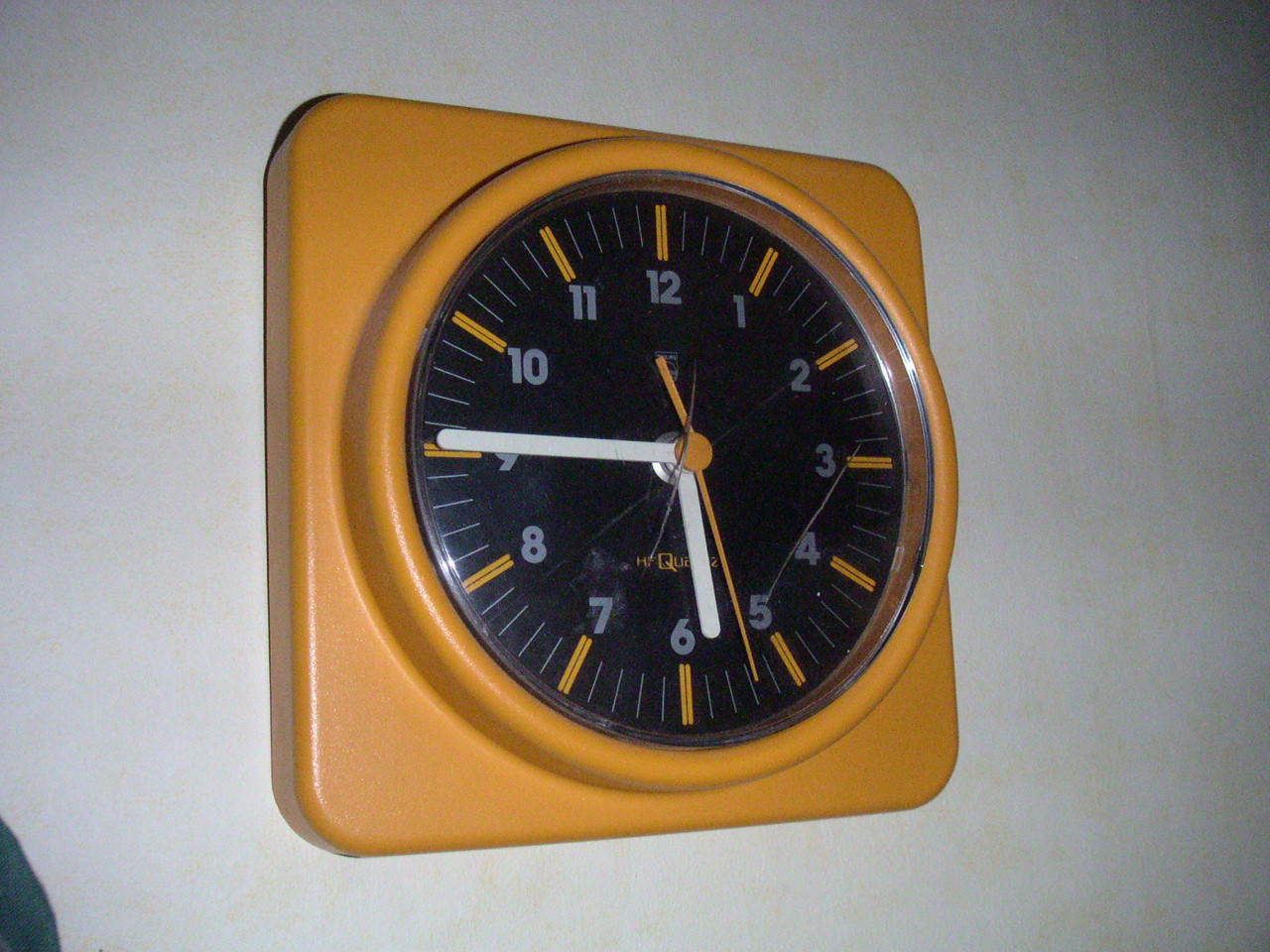This photograph features a distinctive wall clock mounted on a stark white wall. The clock has an orange plastic frame that forms a square with gently rounded corners. In the center of this square frame is a raised round bezel made of the same plastic material. The clock face is black and is encased in clear plastic, which has two visible cracks running horizontally from approximately 1 o'clock to near 7 o'clock and from 3 o'clock to near 5 o'clock.

The clock’s time reads 5:45, indicated by white hour and minute hands, and an orange second hand, matching the frame. The numbers on the clock are gray and range from 1 through 12, positioned beneath thin horizontal and vertical orange hour markers. There are subtle light gray lines marking the minutes between the orange hour indicators. The clock operates with quartz movement and presents a sleek, modern design despite the superficial damage on its face.